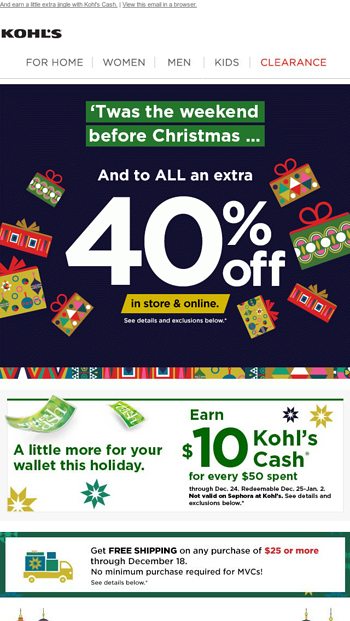This is a promotional page for the store Kohl's. At the center of the page is a large advertisement set against a black background, featuring prominently illustrated gifts that surround a bold, white text displaying "40% off" in sizable font. Above the central graphic is a green banner with the festive message, "'Twas the weekend before Christmas and to all an extra 40% off in-store and online." In the upper left-hand corner of the page, the Kohl's logo, presented in bold black font, anchors the layout. Beneath the logo, a navigation menu includes options for Home, Women, Men, Kids, and Clearance, with "Clearance" highlighted in red and the remaining text in dark gray. Directly below the 40% off ad, another advertisement invites customers to enjoy extra savings with the message, "A little more for your wallet this holiday. Earn $10 Kohl's Cash," written in green text and accompanied by star illustrations and visuals of Kohl's Cash coupons.